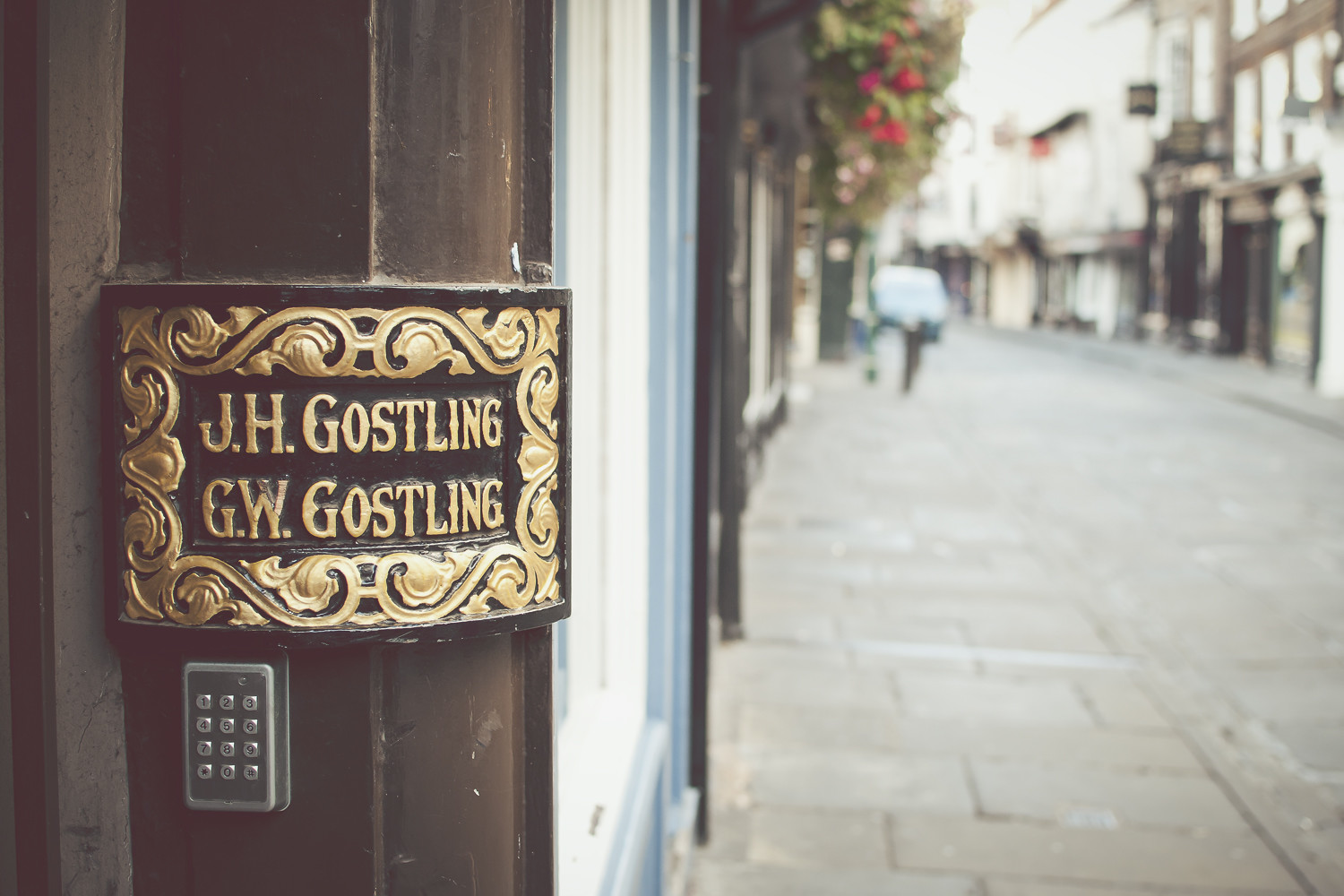The photograph captures a detailed street scene in an older part of town. The stone-paved street features various storefronts with a notable white building accented with dark wood panels on the left side of the image. Prominently displayed on this building is an ornate sign with gold and burgundy details, bearing the names "J. H. Gosling" and "G. W. Gosling" in gold lettering. Directly below the sign is a gray metal keypad with numeric buttons and additional star and hashtag keys. The background shows tall, aged buildings to the right, and a blurry blue car is visible down the stone street. Additionally, a hanging planter with greenery and red flowers adorns one of the storefronts on the right side, adding a touch of color to the scene. The image focuses on the intricately designed sign, while people in the foreground and background appear blurred, emphasizing the historic charm of the location.